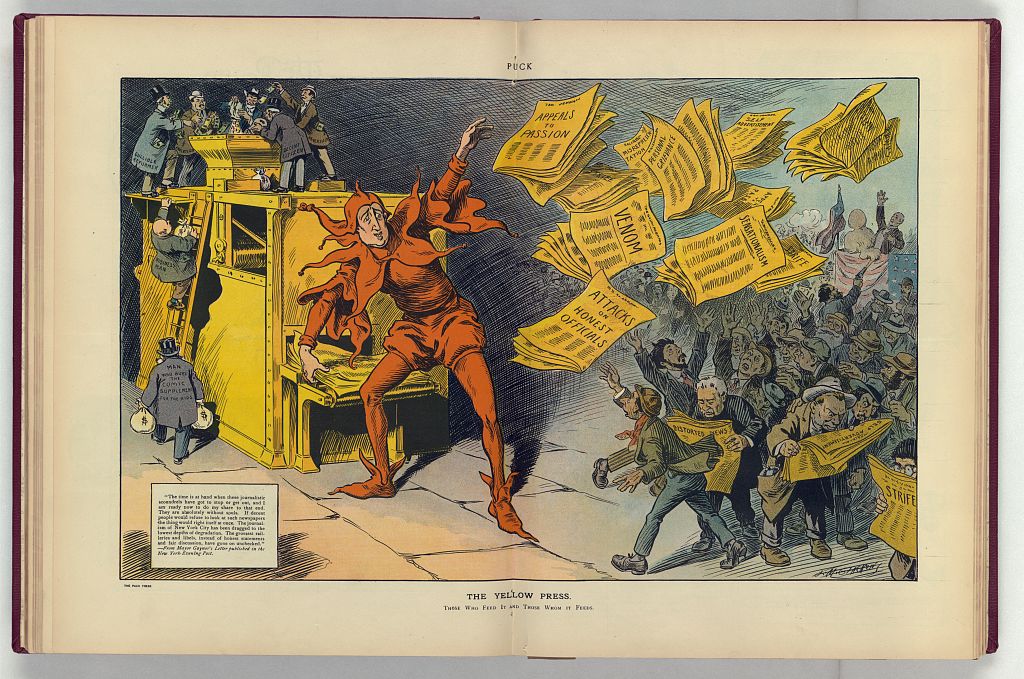This image is a detailed, politically charged cartoon spanning the open pages of a book, specifically from the publication "Puck". At the top, the word "Puck" is prominently displayed. Central to the image is a tall figure dressed as a court jester in a red outfit, symbolizing deceit and manipulation. This jester is energetically throwing yellow newspapers—bearing sensationalist titles like "Venom," "Appeals to Passion," "Attacks on Honest Officials," "Sensationalism," and "Misrepresentation and Strife"—towards a crowd of ordinary, downtrodden people, some in rags, who eagerly grab these papers.

The left side of the image features a large yellow printing machine, representing the yellow press. Small businessmen, depicted as midgets, climb this machine with money bags, feeding their wealth into its intake bin. At the bottom of the machine, freshly printed yellow newspapers emerge, illustrating the corrupting influence of their money. 

In the background, an American flag atop a podium and a preacher with his hands raised to the sky can be seen, adding to the satirical nature of the cartoon. The entire scene underscores the corrupt cycle of sensationalist media fueled by financial interests, preying on and manipulating the public. At the bottom of the image, the text reads "The Yellow Press: those who feed and those whom it feeds," summarizing the critical message of this intricate political commentary.